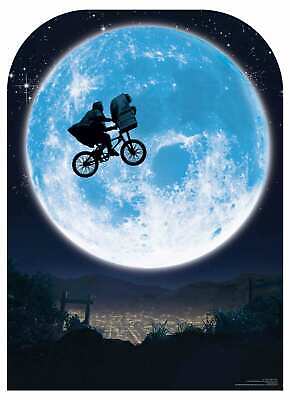The image is a digital screenshot from the iconic 1982 movie, *E.T. the Extra-Terrestrial*. Dominating the upper portion is a large, vividly blue moon. Silhouetted against it is the memorable scene of a young boy named Elliot riding a levitating dirt bike, with an extraterrestrial named E.T. in the basket on the handlebars. This scene is famously used on the logo for Amblin Entertainment, directed by Steven Spielberg. Elliott, dressed in Halloween attire to disguise from federal agents pursuing them, rides from the left to the right of the image. The backdrop below the moon features a well-lit cityscape of a Southern California town and some shrubbery, with parts of a fence and vegetation visible. The colors are primarily light blue, white, and black, with hints of yellow and green, though the typical gray-white moon appears strikingly blue in this depiction. The iconic image captures the magical moment of the bike ride crossing the moon, set against a starry night sky.